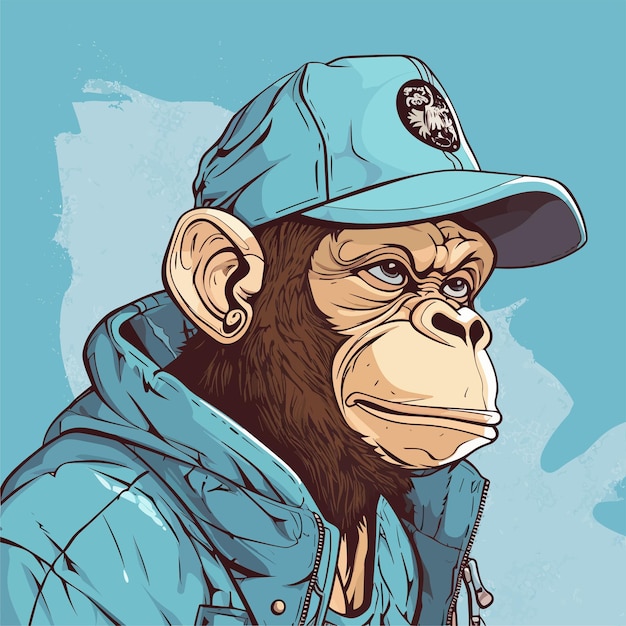This is a detailed vector illustration of a brown-furred ape, specifically a gorilla, with a tan-colored face and ears. The gorilla is donning a sky blue baseball cap featuring a black circular badge, though the design on the badge is unclear. Complementing the cap, the gorilla is also wearing a sky blue puffer jacket. The background consists of varying shades of sky blue, creating a subtle yet cohesive backdrop. The gorilla is depicted in a tough, stoic manner, exuding a hip, modern vibe reminiscent of NFT artwork, as it gazes off into the distance. The artwork's style is characterized by sharp, clean lines without blending, aligning closely with pop art aesthetics.